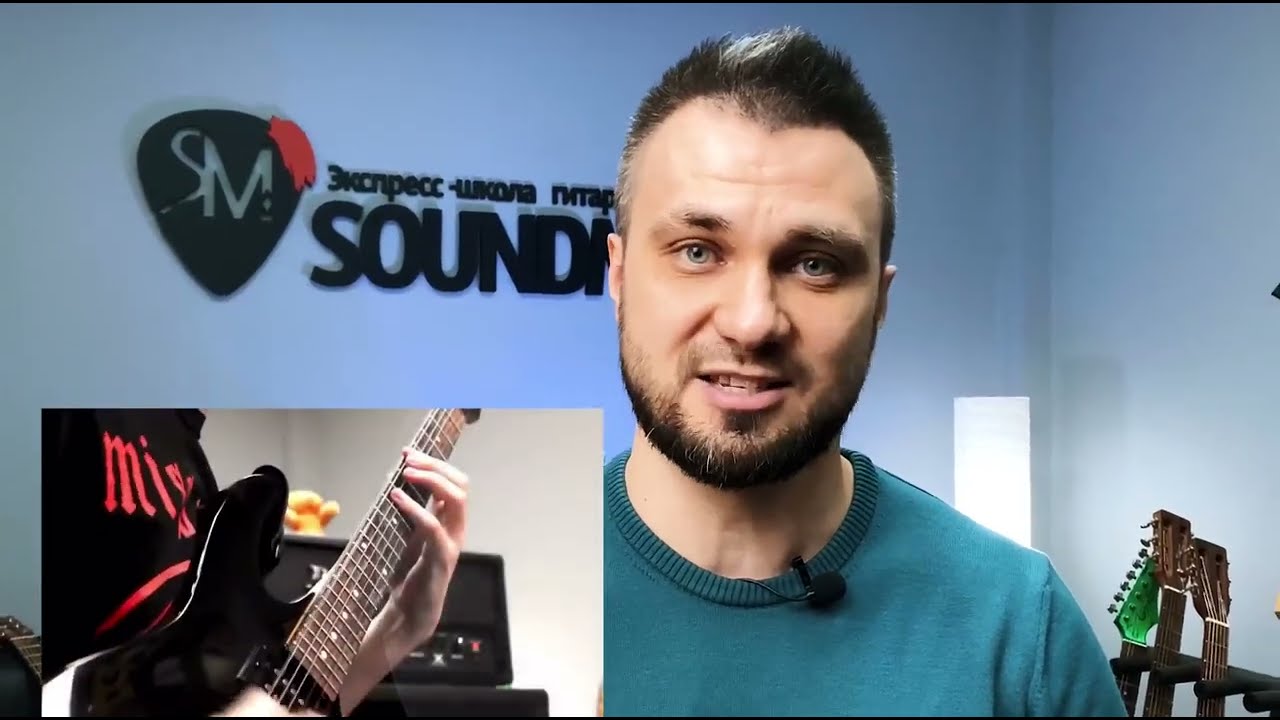The image appears to be a screenshot from a video advertisement or a tutorial video, possibly intended for platforms like YouTube or Twitch. The focal point is a man centered in the image, who has spiky black hair with a graying spot on top, accompanied by a dark goatee. He looks like he's addressing the camera, possibly giving a presentation, with a microphone clipped to the collar of his turquoise or light teal sweater. Behind him, the walls are light blue, and a logo, resembling a guitar pick with the letters 'SM' inside, is prominently displayed. Beneath this logo, there is some text in a foreign language, partially obscured by the man's head, with the word "sound" being visible. To his right, there are three guitar necks resting on a stand. In the bottom left corner of the image, there's a rectangular inset showing a person in a black shirt playing an electric guitar. The scene is clearly indoors, and the various visual elements suggest a well-equipped setting for either guitar lessons or music-related content.